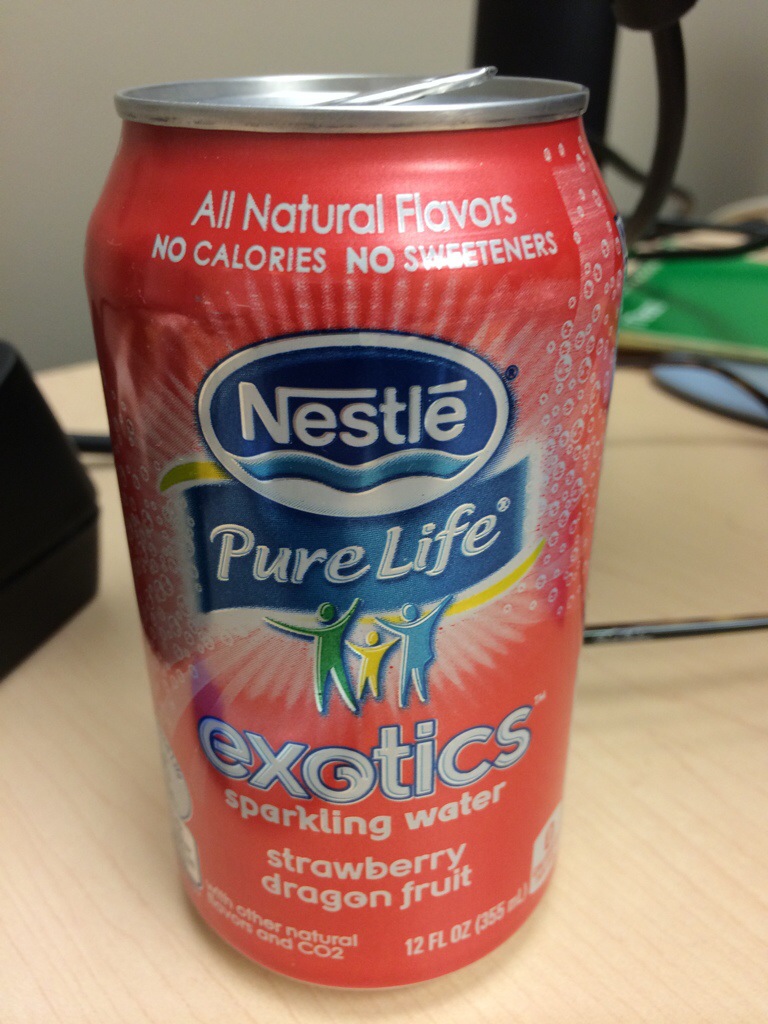This photograph features a can of sparkling water positioned on a light beige wooden desk. The sleek aluminum can is adorned with a silver top and lid. The backdrop of the can displays a light coral pink hue, providing a vibrant contrast. Various text elements, primarily in white, indicate flavors and branding: "Exotic Sparkling Water," "Strawberry Dragon Fruit." At the top of the can, the Nestlé logo is prominently displayed, accompanied by the words "Pure Life" beneath it. Below this, three stick figures in green, yellow, and blue add a playful touch. In the background, an assortment of cords and folders adds a touch of everyday clutter, providing context to the setting.